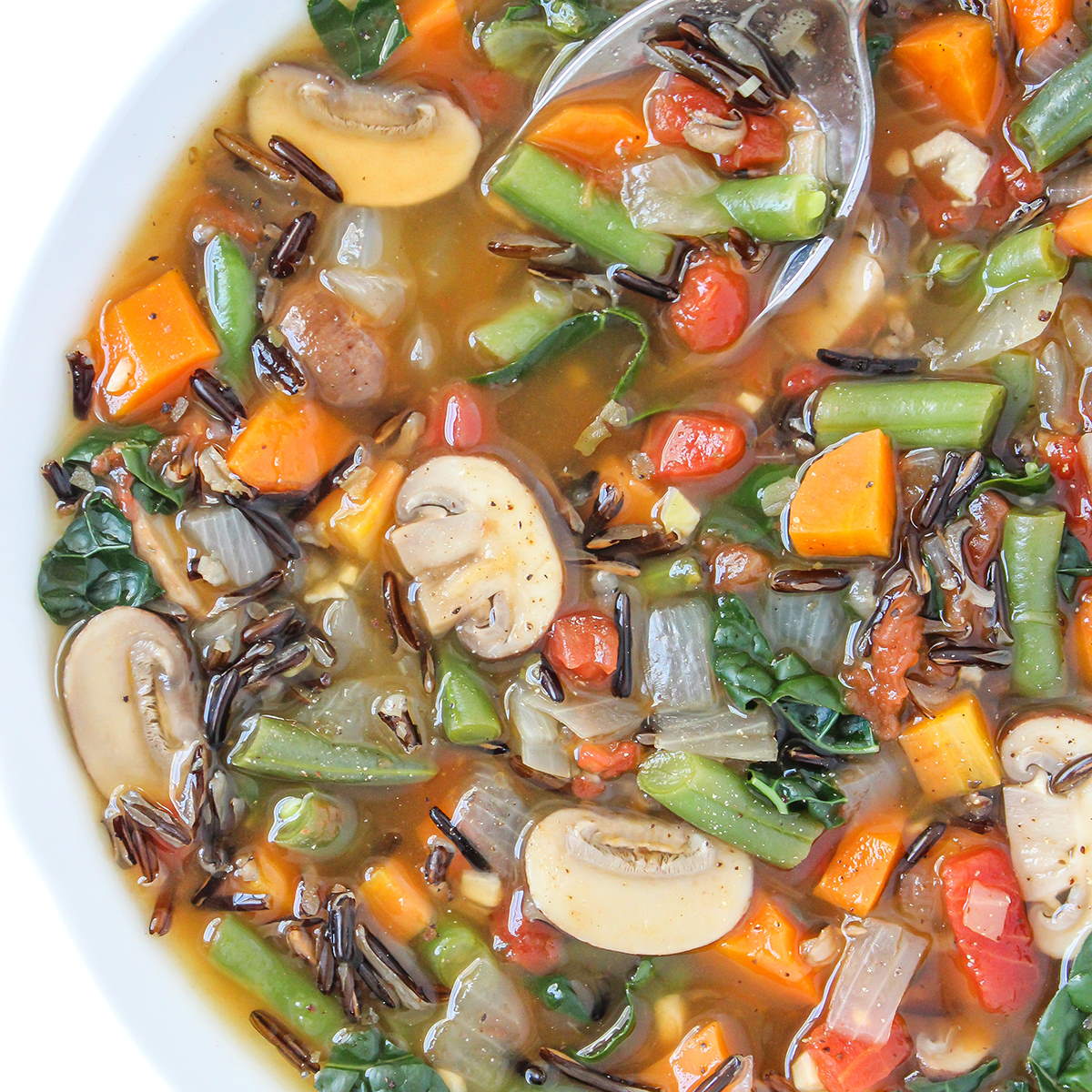The image captures a professionally taken, full-color photo of a bowl of hearty vegetable soup. The soup is served in a white bowl, seen from an angle that reveals about three-quarters of it, with the top, bottom, and right sides cut off, making it appear vertically rectangular. There's no discernible background as the focus is entirely on the bowl of soup. The broth, a rich brownish-red color, is filled to the brim with an assortment of vibrant vegetables including mushrooms, green beans, carrots, diced tomatoes, and onions— the latter of which appear nearly transparent from thorough cooking. Alongside these, there's also evidence of spinach leaves, celery, and possible hints of garlic. A spoon, positioned at the upper right of the bowl, is either silver or clear plastic and holds a variety of the soup’s ingredients, as if in the process of being lifted for a bite. The overall presentation is colorful and inviting, capturing the essence of a nutritious, vegetable-packed meal.